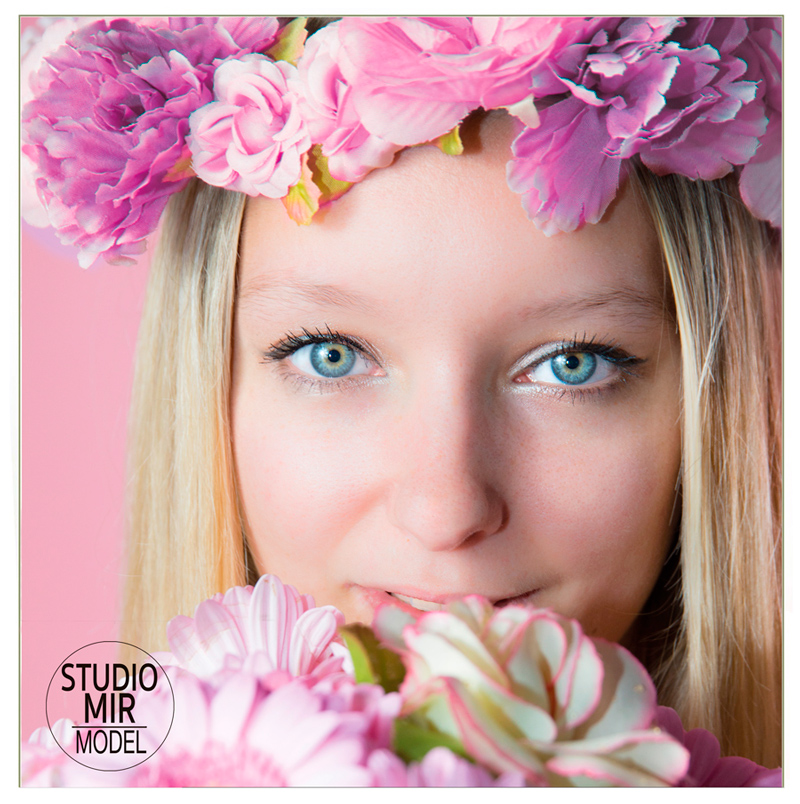This highly stylized, professional close-up portrait features a beautiful young blonde woman, likely in her late teens or early 20s, set against a vivid pink background. Her blue eyes, accented with mascara for a fresh, natural look, gaze directly into the camera. Her long, straight blonde hair is adorned with a crown of large pink and white flowers that extend over the top couple inches of her forehead. She holds a matching bouquet of pink and white flowers high enough to obscure the lower inch or two of her face, including her bottom lip and chin. The close crop of the image focuses entirely on her face and flowers, making her slightly smiling expression and blue eyes the central point of attention. In the lower left-hand corner, the image bears the branding "Studio Mir Model" within a circle in a tall, block text format.